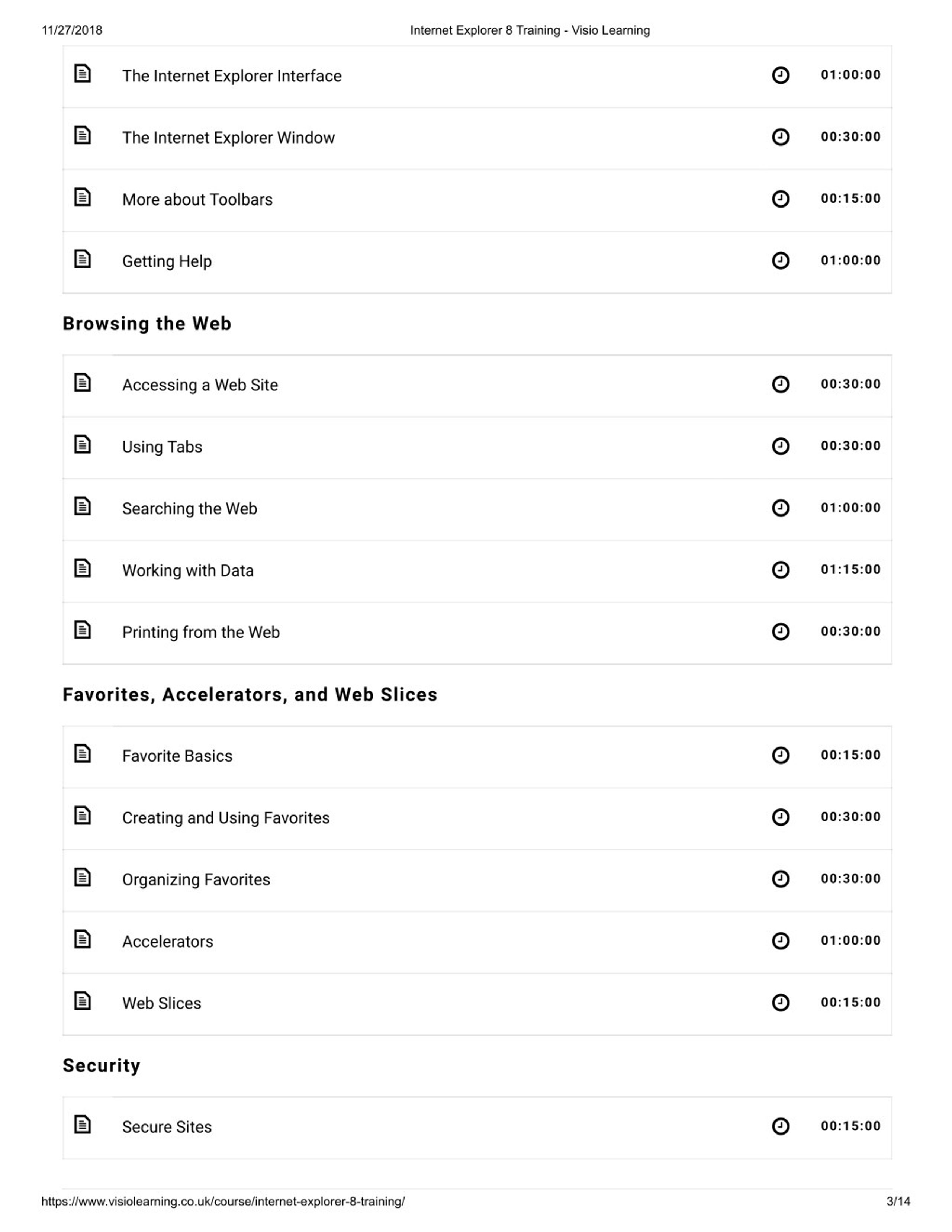**Caption:**

This screenshot features a structured training menu for "Internet Explorer 8 Training" provided by Viso Learning, dated 11-27-28. The menu is meticulously organized into sections, with specific topics listed alongside their respective durations.

At the top, the header prominently reads "Internet Explorer 8 Training, Viso Learning." To the left, the date "11-27-28" is noted.

The first column contains training topics detailed with a page icon on the left. The topics include:
- **Internet Explorer Interface** (1 minute)
- **Internet Explorer Window** (30 minutes)
- **More About Toolbars** (15 minutes)
- **Getting Help** (1 hour)

Following these, the title "Browsing the Web" appears, introducing subtopics such as:
- **Accessing a Website**
- **Using Tools**
- **Searching the Web**
- **Working with Data**
- **Printing from the Web**

Next, the title "Favorites, Accelerators, and Web Slices" is bolded. This section encompasses:
- **Favorite Basics**
- **Creating and Using Favorites**
- **Organizing Favorites**
- **Accelerators**
- **Web Slices**

Further down, the bolded title "Security" is listed, with a single section titled:
- **Secure Sites**

At the very bottom of the image, there is a website address, and in the bottom right corner, the notation "3 of 14" indicates the current page out of the total training material.